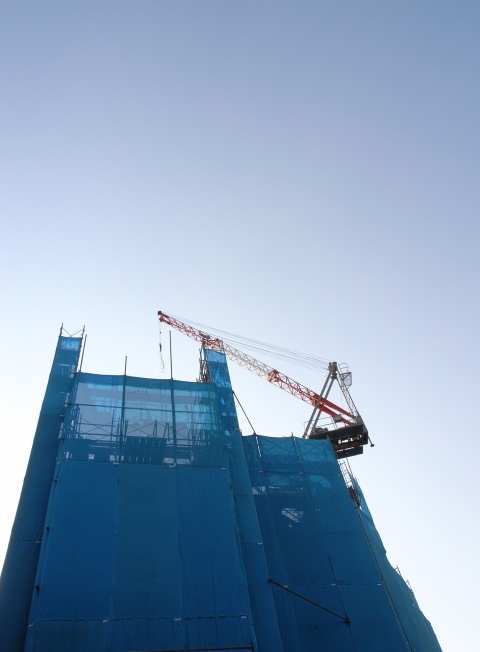This image captures the view from the ground up of two buildings under construction against a backdrop of a bright, cloudless, blue sky. The larger building on the left, primarily dark blue, is still being built and features metal scaffolding and some completed windows. Dominating the scene is a towering red metal crane with a long boom and a hook at its end, extending high above the building. The crane also includes a black walkway section where a person can be seen controlling it from a bucket-like area. To the right, a slightly smaller building features a black antenna near the bottom. Overall, the scene epitomizes the hustle of construction activity on a clear daytime.